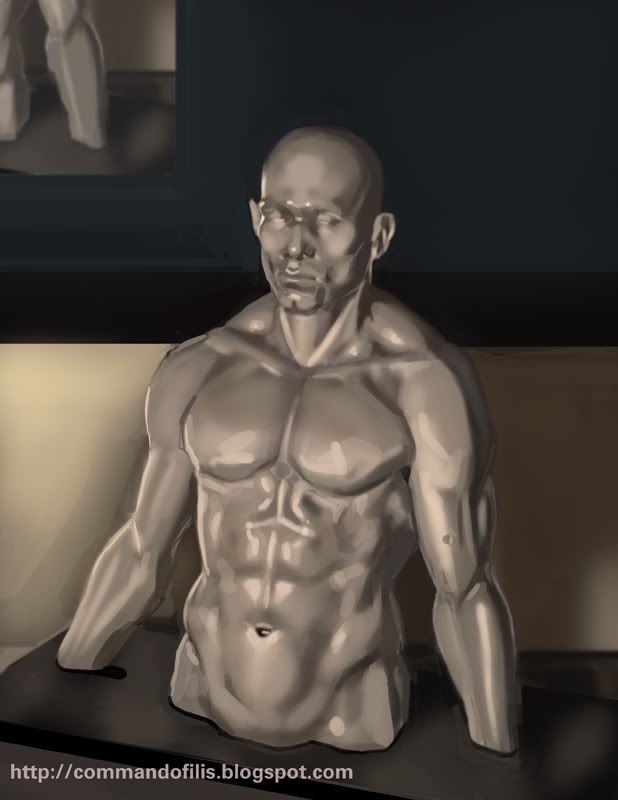The image depicts a highly detailed, silver mannequin of a muscular man, featuring chiseled arms, broad shoulders, and a wide chest. The mannequin is positioned looking off towards the left, with its forearms extending forward, attached to a black stand. The figure is headless and handless, with a focus on its anatomically detailed upper body. In the center of the image, there is a prominent "PhotoBucket" watermark consisting of circular designs and a white banner that reads "Protect more of your memories for less!" In the bottom corner, the website "http://commandofeelings.blogspot.com" is visible against a beige background, blending seamlessly with the black wall behind.